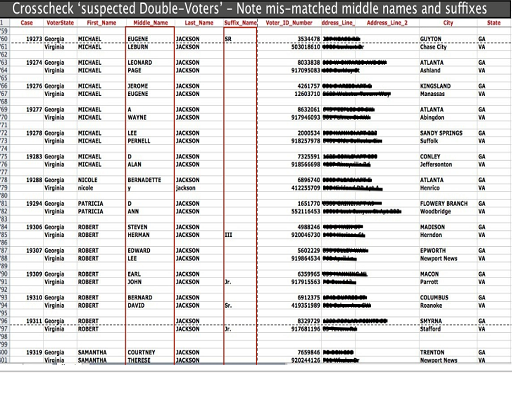The image depicts a spreadsheet titled "Cross-Check Suspected Double Voters - Note Mismatched Middle Names and Suffixes." The spreadsheet lists details of suspected double voters with headings including case numbers, voter states, first names, middle names, last names, suffixes, voter ID numbers, addresses, cities, and states. The rows are numbered from 59 to 101, with space between every two entries. The first names are primarily Michael, Patricia, Robert, and Samantha, all sharing the last name Jackson. Some information columns are blacked out, indicating the focus on potential duplicate voters in states such as Georgia and Virginia, with cities listed including Atlanta, Sandy Springs, Flowery Branch, Madison, and Macon.